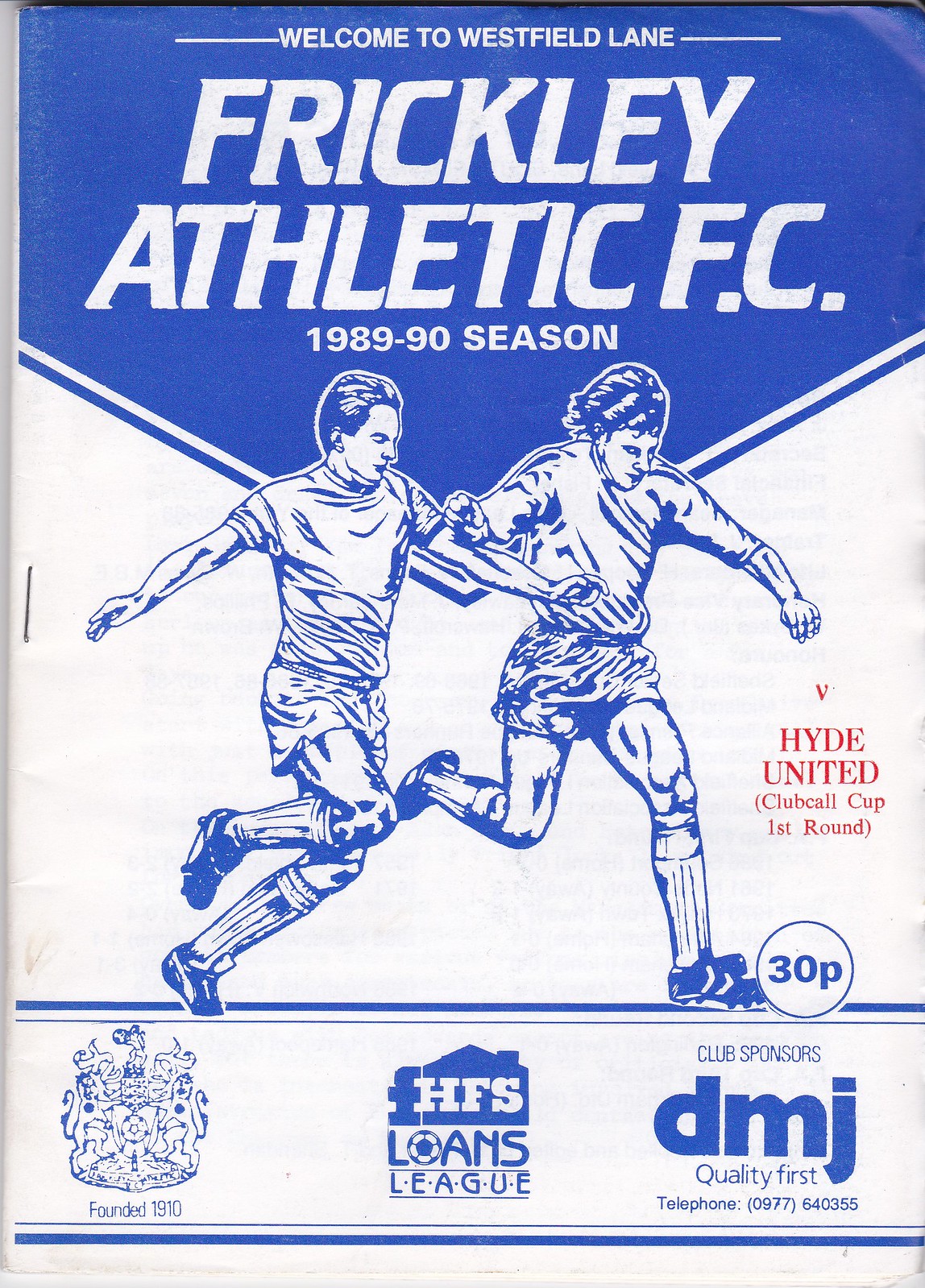The image depicts a detailed notice about a football match, prominently featuring a textured blue background. At the top, in white text, it announces, "Welcome to Westfield Lane, Frickley Athletic FC, 1989-1990 Season." Just below, an illustration shows two football players in the midst of a game, vying for a ball. To the right of this drawing, red text labels the event as the "Hyde United Club Call Cup 1st Round." Next to the players, a circle indicates the price, "30p." The bottom section includes various logos: on the left, a logo accompanied by the text "Founder 1910"; in the center, the HFS Loans League logo; and on the right, the Club Sponsors, "DMJ Quality First," along with a telephone number, "09776 40355."